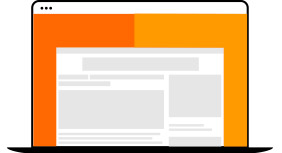This is a detailed illustration of a contemporary computer, created through digital means. The image is outlined in black, clearly depicting the computer with a pronounced keyboard that protrudes, suggesting it might be either a laptop or a monitor resting on a shelf. At the top of the screen, a white bar stretches horizontally from the left side to the right, adorned with three distinctive dots in the upper left corner.

Beneath this white bar, the screen features an upside-down L-shaped figure, which extends horizontally from the left and reaches the midpoint of the computer display. The vertical part of this shape continues down to the bottom of the screen. Mirroring this, on the right side, is another upside-down L-shaped figure, this time in orange, spanning from the center of the screen to the right edge and also stretching vertically to the bottom.

The space between these two shapes forms the computer's main display area, entirely white, with some indistinct, light gray images faintly visible. The detailed information on the screen appears to be obscured or greyed out, adding a layer of intrigue to the overall design.